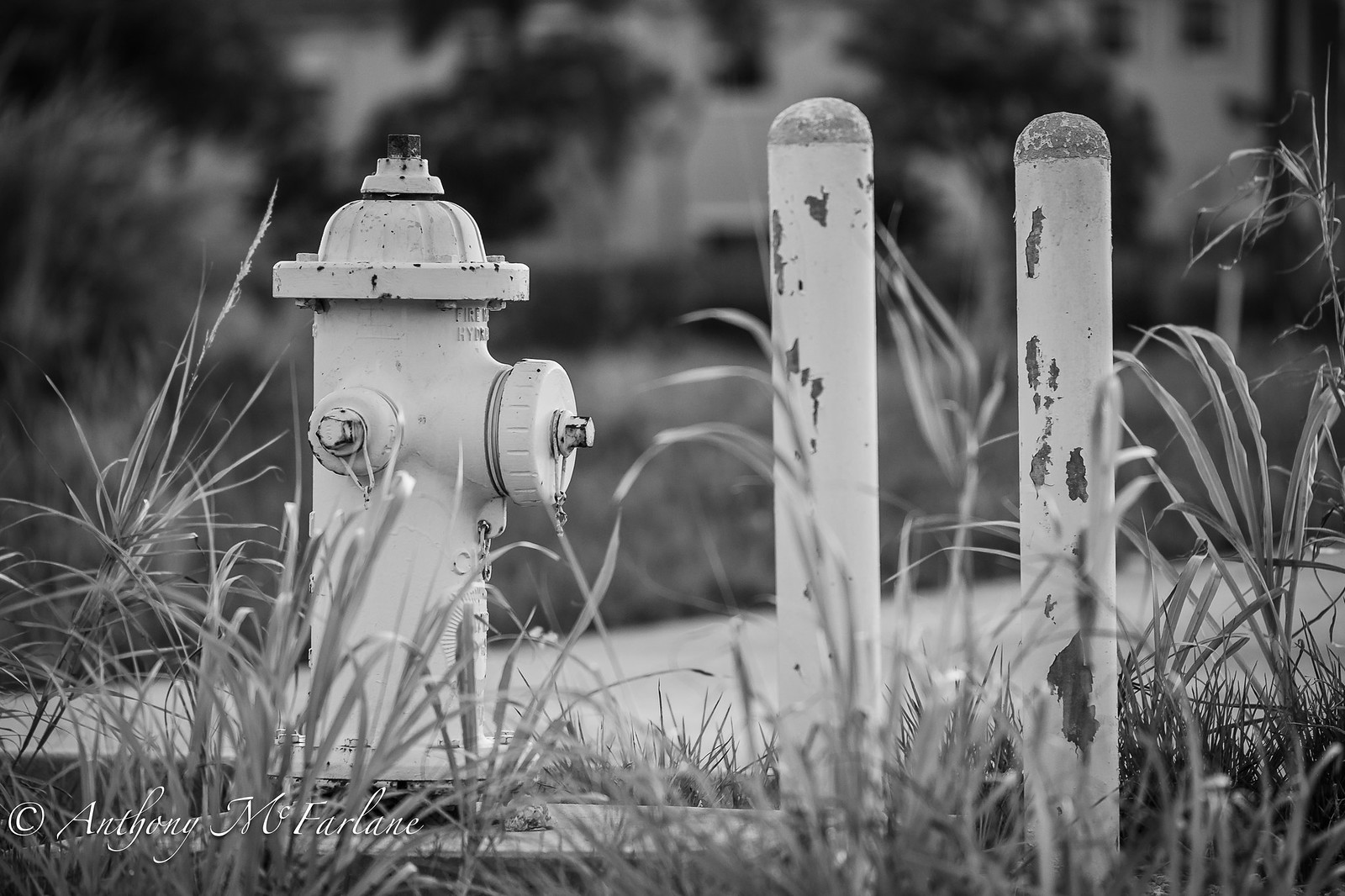A black-and-white photograph prominently features a pale fire hydrant on the left side, accompanied by two weathered, white or light-colored poles of similar height to the right. The foreground is overgrown with sporadic tall grass and weeds, covering parts of the hydrant and poles. Behind this focal setup, a gray sidewalk extends into the distance, marking the midsection of the image. The upper two-thirds of the photo are blurred, revealing only hazy outlines of a large, light-colored building with two stories, characterized by a series of dark, rectangular windows on the second level. Blurry tree branches hang in front of the building, which is bordered by a hedge and a grassy area. Notably, the lower left corner of the image bears a cursive signature, “Anthony McFarlane,” identifying the photographer.